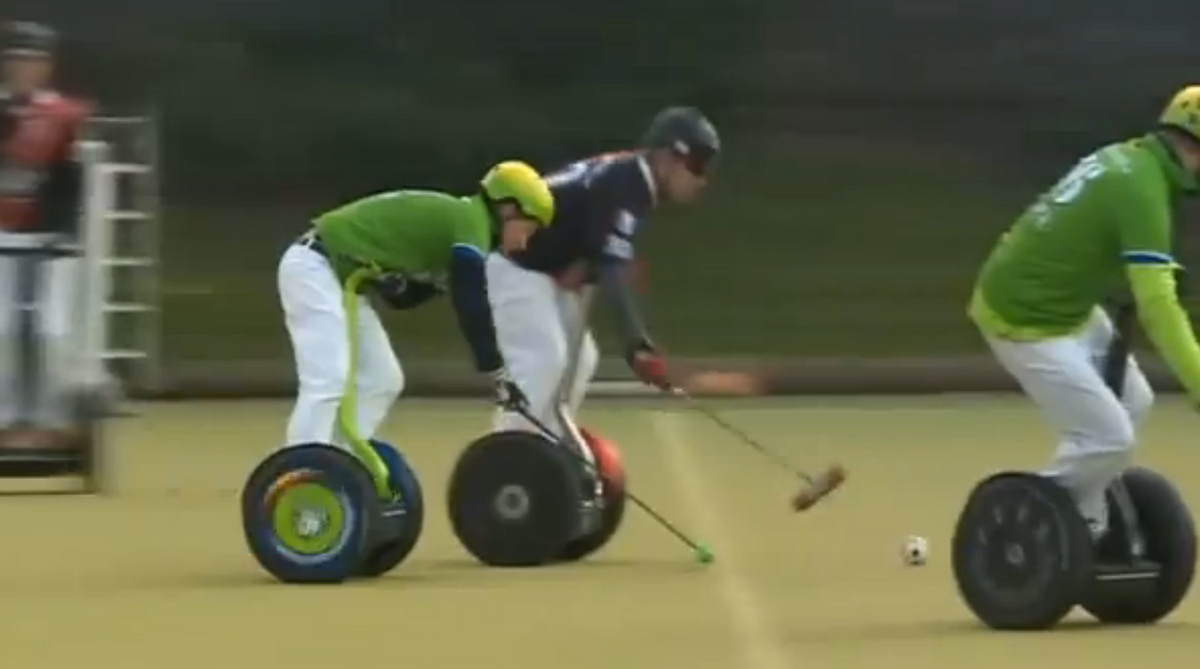This photograph captures a high-speed game that closely resembles polo but played on motorized Segway-like scooters with polo clubs in hand. The scene unfolds on a lush green field, with three main players prominently featured. In the front, a man donned in a green helmet, green shirt, black undershirt, gloves, and white pants rides his two-wheeled device. Just behind him, another player wears a black helmet, a black jersey, and white pants, also maneuvering a similar scooter. To the far right, a third participant, sporting a green helmet, green jersey with a barely visible number '6', light green undershirt, and white pants, is part of this dynamic play. They are all chasing a small ball with a distinct black dot. 

In the blurred background, a figure in a maroon shirt and black hat stands on a platform, potentially serving as a referee. The scene is enveloped in a blur of motion, emphasizing the fast-paced nature of the game and the intensity of the competition.